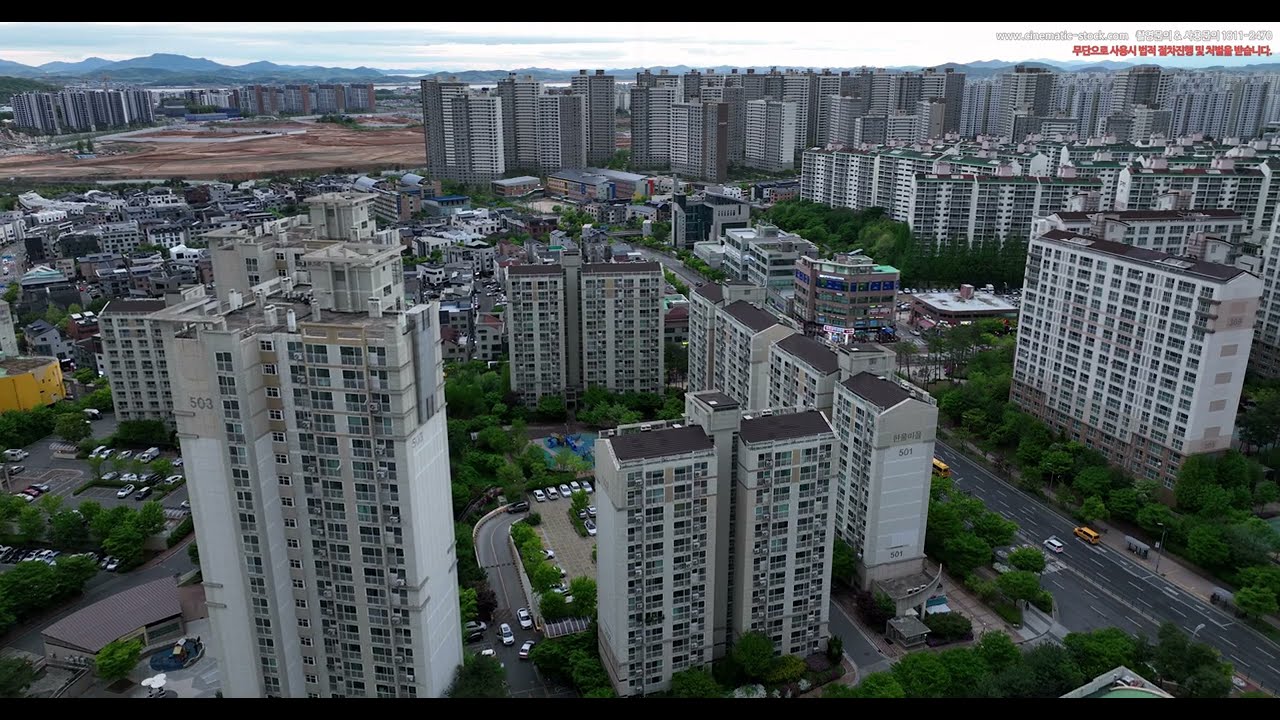This aerial photograph displays a dense urban area featuring numerous tall, identical gray concrete high-rise buildings. The skyline reveals a sprawling cityscape extending to a distant mountain range. In the upper right corner of the image, small, almost illegible white and red text in Chinese characters suggests the photo may have been digitized. The high-rises, reminiscent of apartment buildings in New York, showcase uniform flat facades, numerous windows, and balconies. Trees are interspersed among the buildings, adding greenery to the urban environment. Key details include a road with school buses and various cars, a small courtyard in front of the foreground building marked with the number 503, and a parking lot behind two buildings. A bare dirt area in the far left hints at ongoing construction for additional residential complexes. No people are visible in the scene, which is captured from a high vantage point.